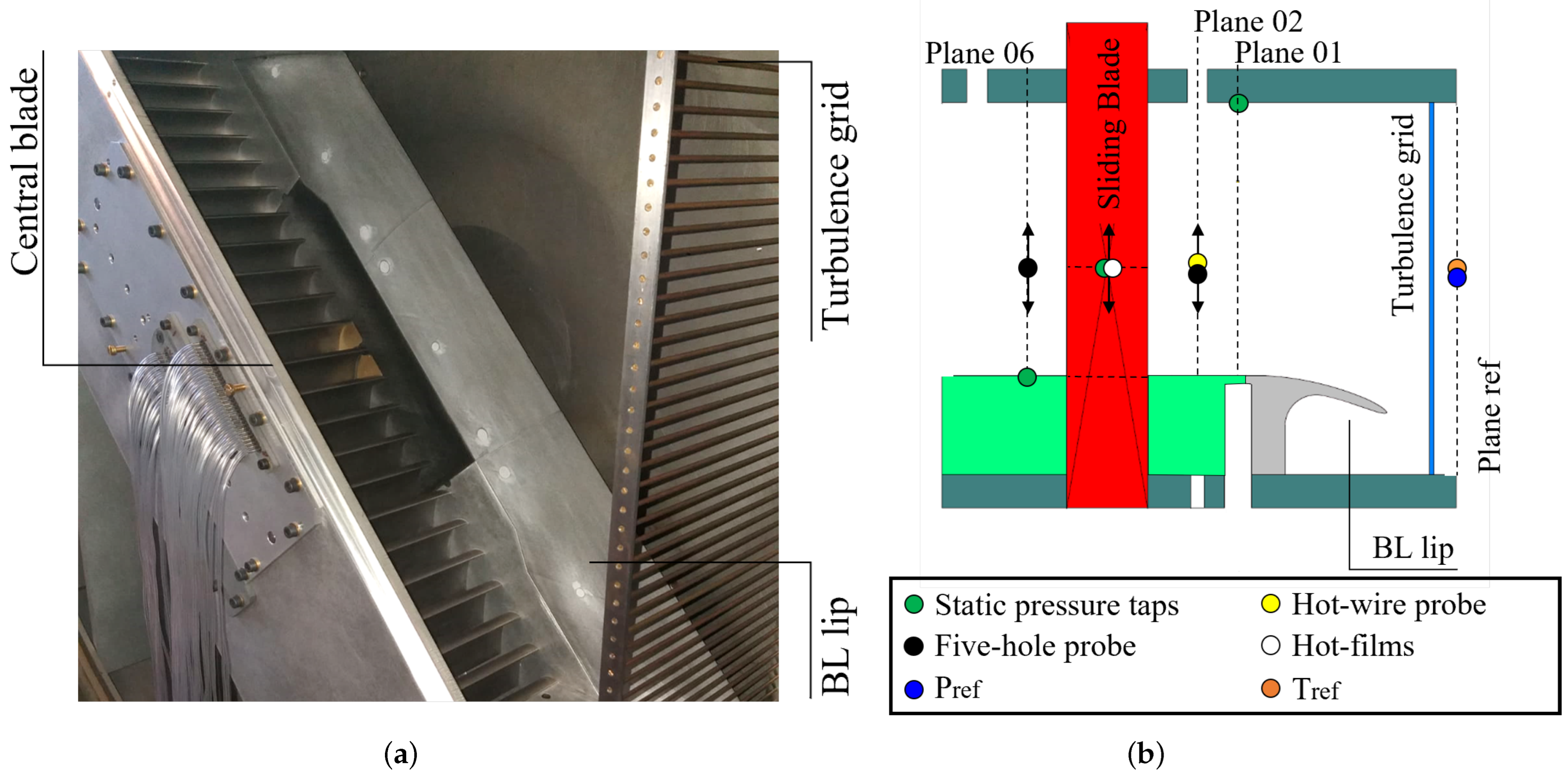This image consists of two sections: a photograph on the left labeled "A" and a detailed scientific diagram on the right labeled "B." On the left, the photograph showcases a metallic structure referred to as the "central blade," which resembles an industrial component, possibly an HVAC or furnace system. Visible elements in the photo include a series of cables emerging from the left side of the central blade, a "turbulence grid" on the right, and the "BL lip" at the lower part of the structure. 

The diagram on the right complements the photograph by providing a schematic overview with precise labeling and color coding. It features a large red rectangle labeled "sliding blade" within a green rectangle, alongside various "plane" references such as plane 06, plane 02, and plane 01. The right side of this diagram also matches the photograph's depiction of the turbulence grid and BL lip and includes additional labels like "plane ref." 

Below the diagram is a legend that defines the color-coded elements: green for static pressure taps, black for a five-hole probe, blue for P-ref, yellow for a hot wire probe, white for hot films, and orange for T-ref. The comprehensive labels and legend suggest this image is part of an industrial or scientific report, illustrating the components and measurement points of a technical system.